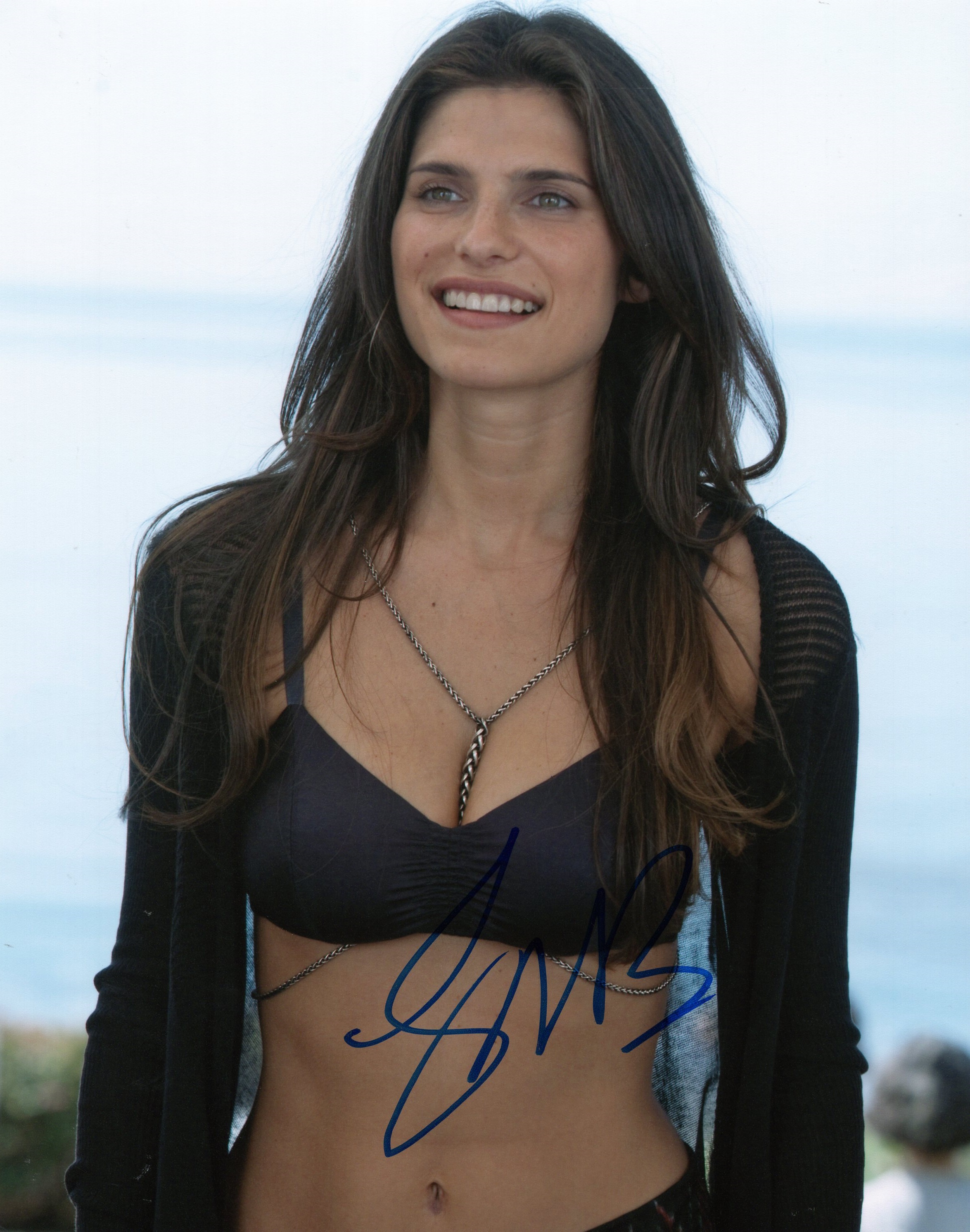This image features a beautiful woman with long, dark brown hair cascading down to her chest, accentuating her striking hazel-green eyes. She exudes a radiant smile, looking towards the left side of the frame, reminiscent of a model's poise. Dressed in a black two-piece bathing suit, she pairs it with a matching black cover-up that drapes over her arms. Around her neck, she wears a long silver chain necklace. The background offers a blend of a white-blue sky and faint, blurry figures, with hints of greenery in the lower corners. Adding a personal touch, the woman has signed the image with a blue magic marker, although the signature is not legible.